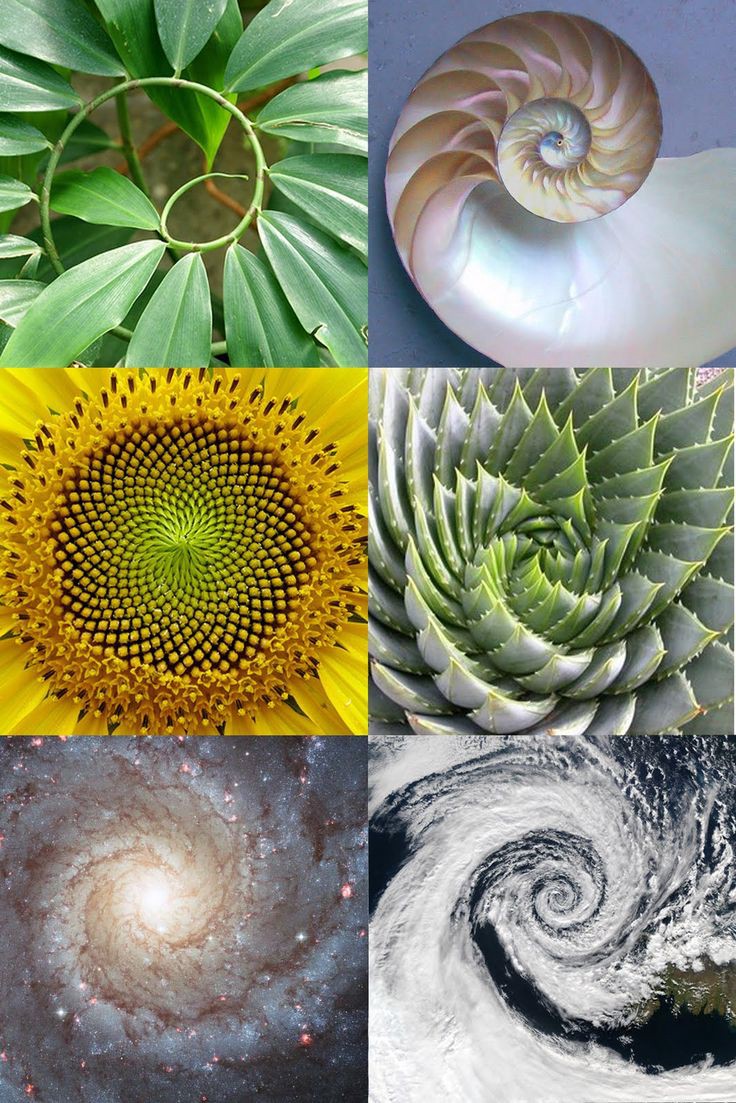The image is a portrait-oriented collage comprising six equally sized photographs arranged in a two-by-three grid. Each photograph showcases a natural phenomenon exhibiting a spiral pattern, illustrating the Fibonacci sequence.

- The top left image features a plant with a curling stem spiraling upward, embellished with large green leaves fanning out in a visually striking pattern.
- Adjacent to it, in the top right, is a detailed close-up of a nautilus shell. This shell displays concentric spirals with a gradient from white at the edge, transitioning through beige and orange hues toward the center, set against a dark blue background.
- In the middle row, the left photograph presents a close-up of the central structure of a sunflower. It captures the intricate geometric arrangement of yellow pollen spiraling inward, accompanied by fluffy, pollen-covered sections and snippets of yellow petals around the edges.
- The right middle image zooms in on the top view of a cactus. Its densely packed, triangular leaves are covered in sharp spikes, organized in a mesmerizing spiral pattern with white flesh and green-tinged tips.
- Occupying the bottom left is an image of a galaxy, showcasing a luminous central core with smoky white and grey spirals peppered with bright red specks, suggestive of cosmic dust and stars.
- The bottom right photograph depicts a swirling hurricane as seen from a satellite, with thick bands of white clouds arcing from the bottom left towards the center, framed by dark blue ocean and a small green landmass in the corner.

Collectively, these images illustrate the pervasive presence of spiral patterns in nature, from botanical structures and marine life to astronomical phenomena and atmospheric conditions.